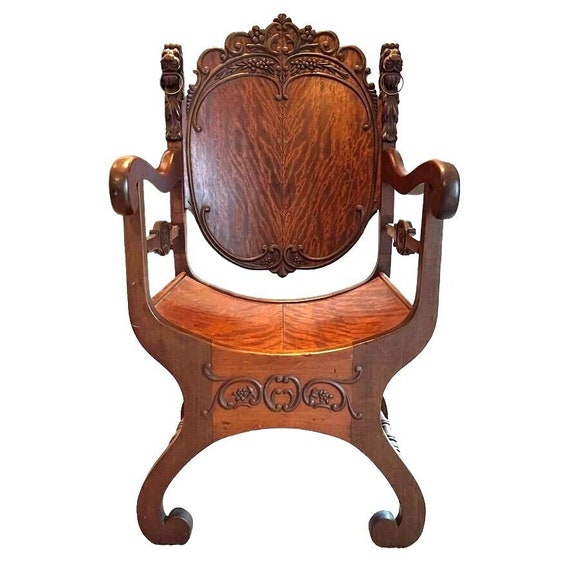This photograph depicts an antique wooden chair, crafted in a style reminiscent of the Tudor or Renaissance era. The chair showcases an intricate design with a dark brown, reddish stain, and includes inlays of lighter-colored wood in the seat, creating a marbleized pattern. The seat is bowl-shaped, complemented by curved, ornate armrests and legs. The front legs feature claw feet that curve into a circular design. The back of the chair boasts a semi-circular, crowned top adorned with waves, triangles, and intricate filigree carvings, akin to a decorative headpiece. The entire piece exudes the high quality and craftsmanship typical of hand-carved furniture that could belong in a palace. The photograph is vertically oriented against a pure white background, emphasizing the chair’s exquisite details and condition.